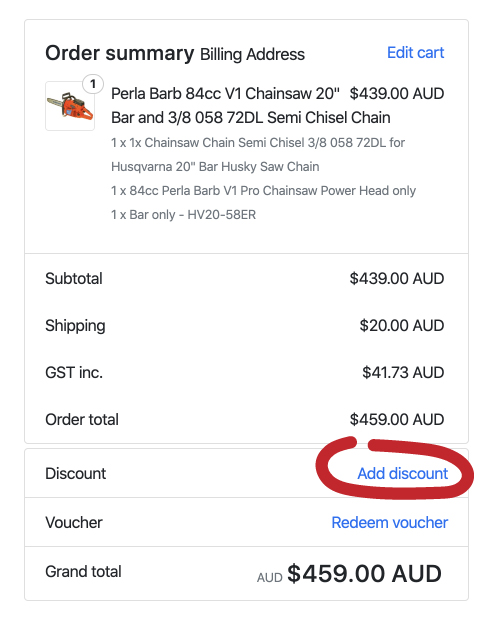This image is a computer-generated order summary for a chainsaw. The focal point of the image is a small square featuring a chainsaw with an attached circle indicating a quantity of one. The chainsaw is described as a "8-4 cc, 20-inch chainsaw," priced at $439 AUD.

Above this section, there is an "Edit Cart" button in blue situated in the upper right-hand corner, allowing the user to modify their order. Below the chainsaw description, additional product information is provided.

The background is predominantly white, and adjacent to the product listing is a detailed summary of the order costs. The subtotal is stated as $439 AUD, with shipping costs amounting to $20 AUD. The GST included is $41.73 AUD, bringing the order total to $459 AUD.

Highlighted in thick red marker is a section for applying a discount, which prominently displays "Add Discount." There is also an option to redeem a voucher by clicking on a blue link.

The grand total at the bottom of the summary underscores the final amount with "AUD $459.00" in large black letters. Overall, the image allows users to review and verify their order and provides clear options to edit the cart or apply discounts before finalizing the purchase.